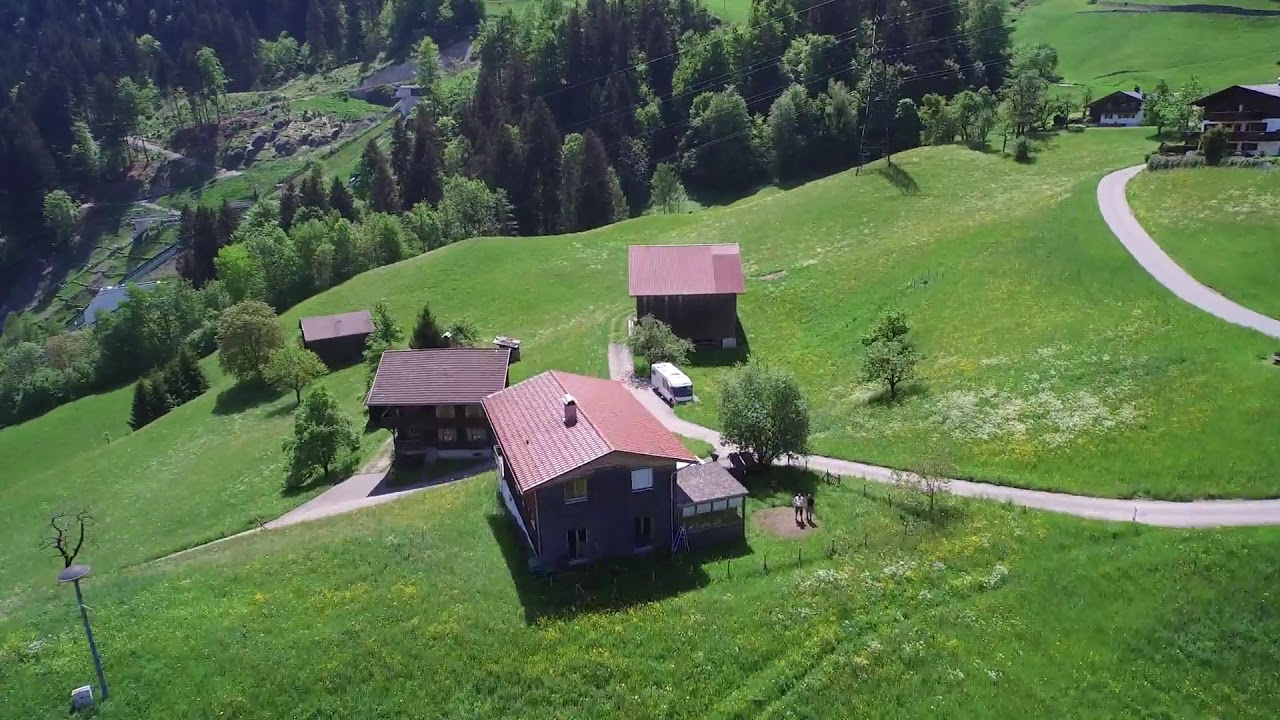This detailed aerial photograph captures a scenic countryside village nestled on a hillside, descending into a lush valley. The central focus is a prominent two-story house with a red V-shaped roof and a chimney, located toward the middle-bottom of the image. This house is surrounded by a large patio or deck and is enveloped by well-maintained green grass. Adjoining the main house are three other structures: one to the left and one to the right of the central house, potentially serving as sheds or detached garages, and another smaller building slightly down the hill to the left.

A cement driveway and pathways connect these buildings, extending toward the right edge of the image and curling upward to meet additional homes situated in the upper right-hand corner. In the image's background, a substantial grove of trees lines the hillside, providing a natural boundary and further enhancing the picturesque setting. The top section of the image showcases the terrain sloping downward, covered with dense trees, rocky areas, and sparse buildings in the distant valley.

Overall, the layout features a cluster of homes with red-burgundy roofs, connected by winding lanes and driveways that integrate seamlessly with the undulating landscape, creating a harmonious blend of rural architecture and natural beauty.